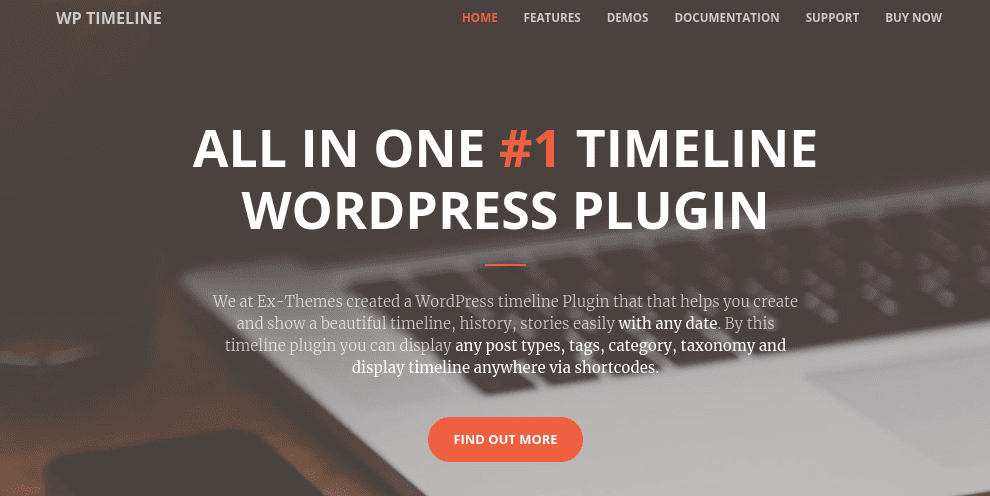This is a screenshot of the homepage of a website called "WP Timeline." At the top left corner, the site's logo is displayed, while at the top right corner, a navigation menu features the following options: "Home" (highlighted in orange), "Features," "Demos," "Documentation," "Support," and "Buy Now" (all in white).

The main image on the page is a somewhat blurry photo of a laptop keyboard with a cell phone placed next to it on the table. The laptop keys are black, while the keyboard and touchpad are silver.

Overlaying this image is a promotional message for the website. It reads: "All-In-One Timeline WordPress Plugin" in bold, white, capital letters. The phrase is interrupted in the middle by the number "1," which is highlighted in orange. Below this headline, a thin orange line separates the main title from a detailed description in smaller print. This text explains that "We at XThemes created a WordPress timeline plugin that helps you create and show a beautiful timeline, history, stories easily with any date. By this timeline plugin, you can display any post types, tags, category, taxonomy and display the timeline anywhere via shortcodes."